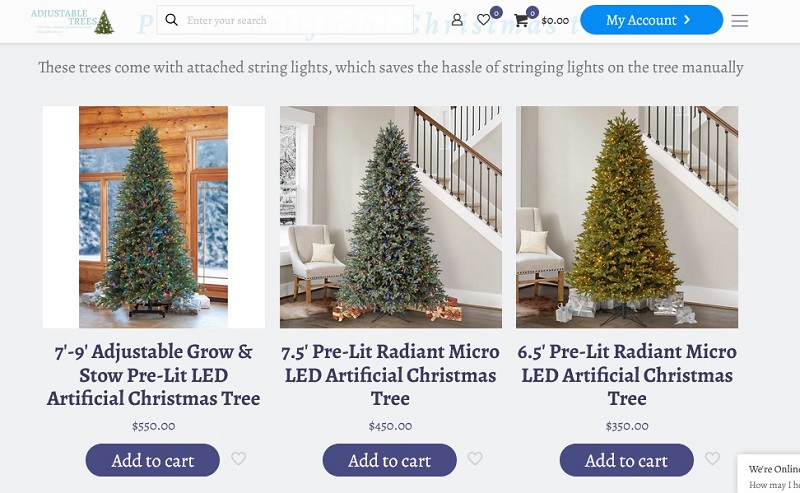This image is a screenshot of a shopping website named "Adjustable Trees." At the very top-left corner of the page, the website's name is prominently displayed, although the smaller accompanying text is unreadable due to its size. To the right of the logo, there is a search bar with placeholder text "Enter Your Search" and an adjacent magnifying glass icon. Further along the top menu, there is a sequence of icons: a profile icon representing the user account, a heart icon with a blue circle indicating zero saved items, and a shopping cart icon also marked with a blue zero, signifying an empty cart. The cart's balance is clearly shown as $0.00. 

Next to these icons is a blue button labeled "My Account," followed by an icon of three horizontal lines that likely opens a sidebar menu when clicked. 

Below the top navigation, there's a text banner explaining that the trees sold on the website come with pre-attached string lights, removing the need for manual installation. 

The main content area presents three images of artificial Christmas trees. The first tree is described as a "7 to 9 feet, Adjustable Grown Stone, Pre-lit LED Artificial Christmas Tree" priced at $550. The second is a "7.5 feet, Pre-lit Radiant Micro LED Artificial Christmas Tree" priced at $450. The third tree is a "6.5 feet, Pre-lit Radiant Micro LED Artificial Christmas Tree" costing $350. Each tree listing has a blue "Add to Cart" button below it, facilitating quick purchases.